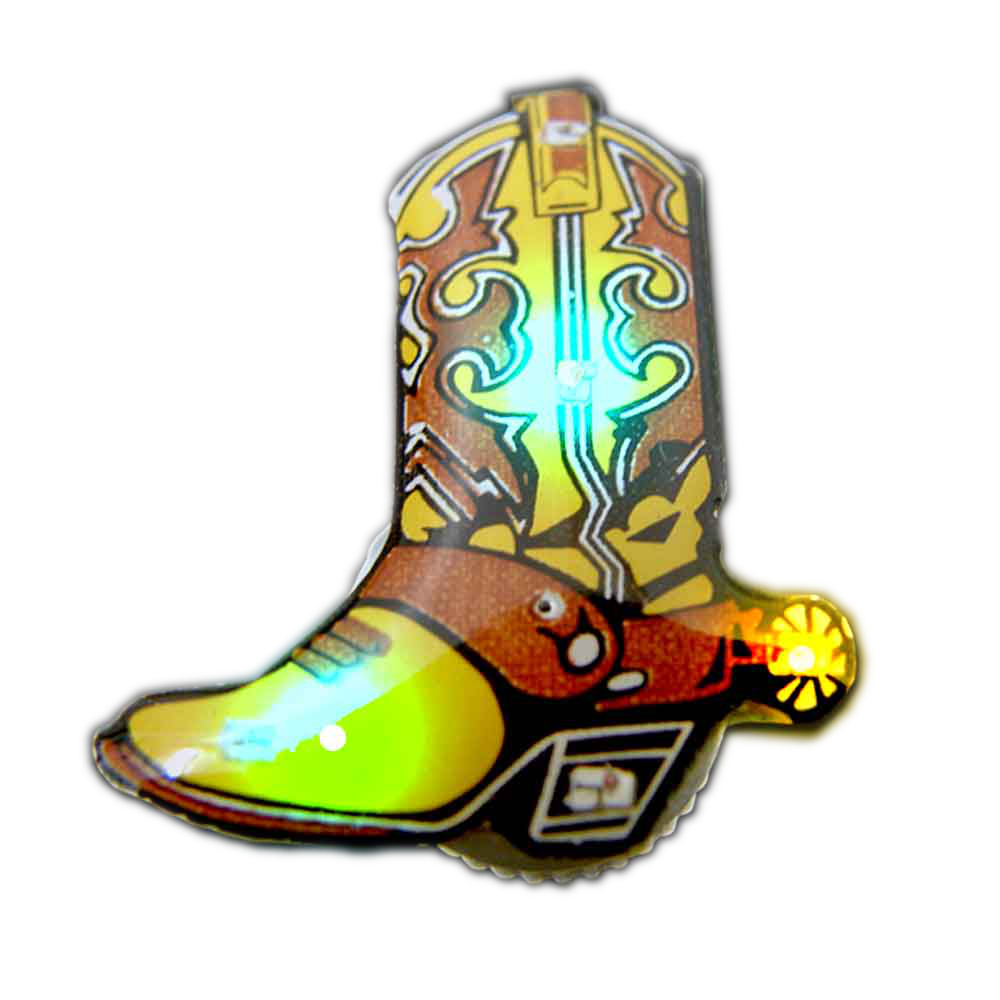This image depicts a small, cartoonish cowboy boot pin or magnet with a high-gloss finish, resulting in severe glare mainly on the left, top, and side of the boot. The boot is primarily yellow with red and brown decorative elements. A red strap extends from the top side to the back, where there is a yellow circle spur without much intricate design. The boot features a brown squiggly design along its upper part, accented by a white outline with a black stripe running down a little rectangle in the center. The front and heel present additional spurs or non-wearable elements that resemble a stirrup or saw blade, contributing to its whimsical appearance. Overall, it captures a vibrant Southwestern aesthetic.